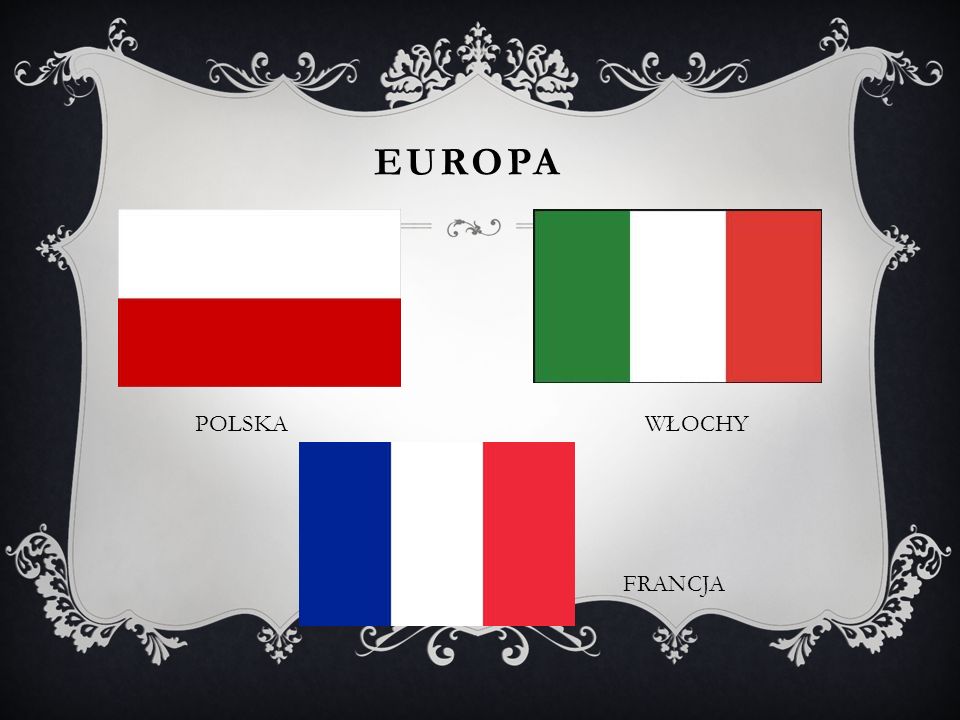The image showcases a solid black background adorned with a silver, elegantly designed emblem that takes up most of the space. At the top, there is a straightforward black title that reads "Europa." Within this emblem are three European flags from Poland, Italy, and France. The Polish flag, positioned on the top left, is depicted as a white rectangle over a red rectangle with the name "Polska" written beneath it. To its right, the Italian flag, featuring green, white, and red vertical stripes, has the label "Włochy" below it. Centrally positioned below these two flags is the French flag, displaying blue, white, and red vertical stripes, with the name "Franca" placed to its right. The text appears to be in languages other than English. A tiny decorative scroll emblem lies nestled between the Polish and Italian flags.